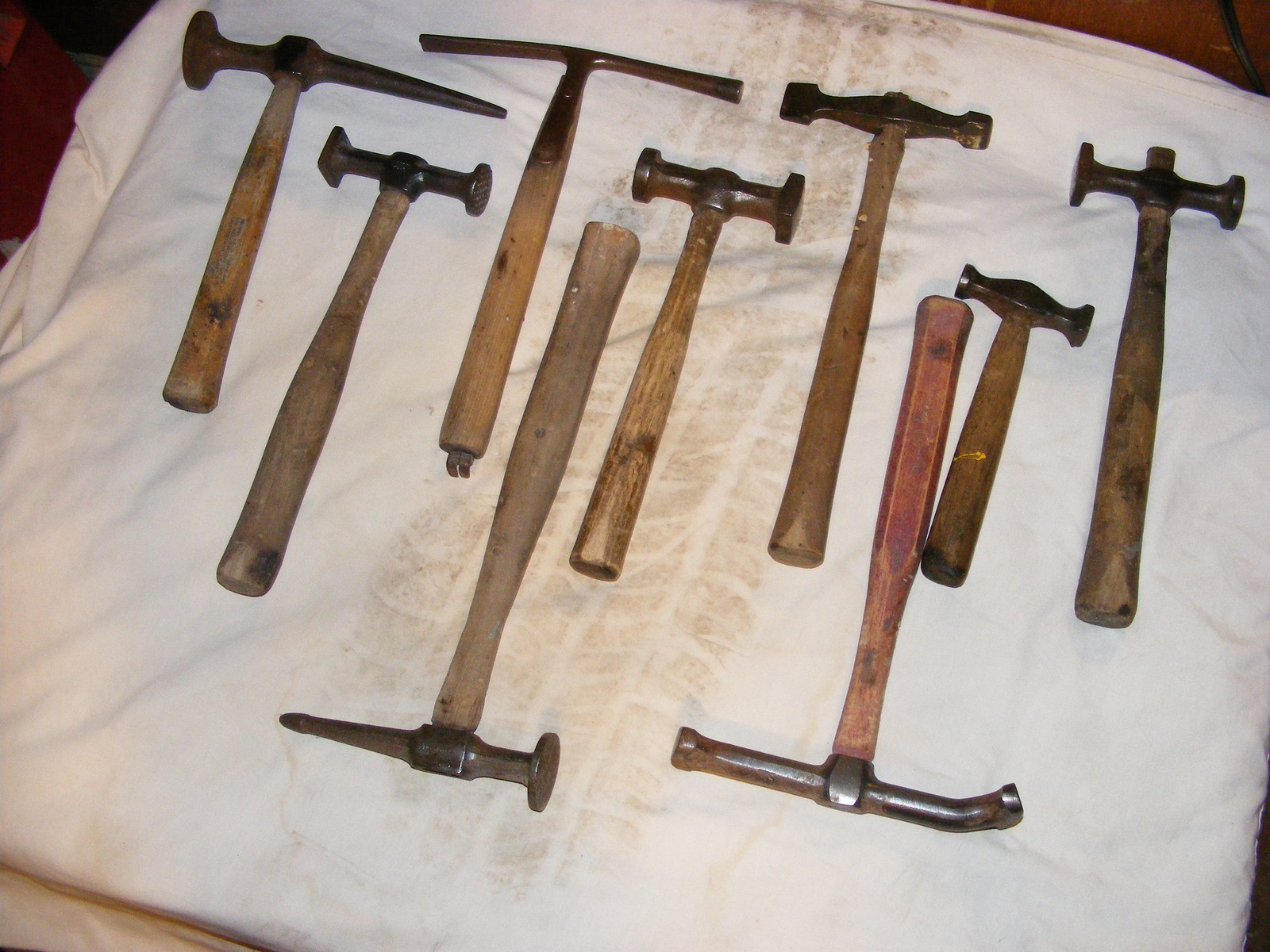The image depicts an assortment of nine hammers and other hand tools laid out on a white sheet, which features what appears to be black or brown tire marks running across its middle. On the left side of the image, a red stand can be seen, while a wood floor and a large black cord are visible in the right-hand corner. The tools include body-working hammers, sledgehammers, and long-peen hammers, each with distinctive metal heads ranging from rounded to square to pointy, and some with unique shapes like a hammer head combined with a small axe head or a pry bar.

The tools primarily have wooden handles, which are rounded at the bottom. Most handles are in shades of brown, looking like traditional wooden handles, and there are two notable exceptions: one with a red handle, reminiscent of redwood, and another with a white handle. Among the hammers, one features a large head on the front and a tapered spike on the back, while another showcases a small head and a thin, flat pry bar on the backside. Additionally, one hammer has a double-headed design. The two hammers set with their handles to the right and heads to the left are silver, contrasting with the chocolate brown and light brown of the other tools.